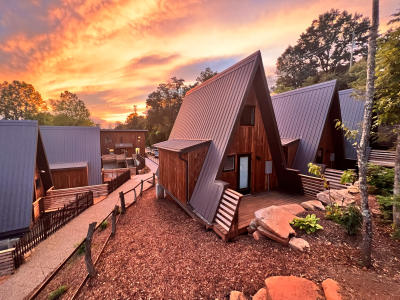This is a horizontal, outdoor photo captured at either sunrise or sunset, showcasing a tranquil, twilight sky painted in hues of orange, pink, and purple, with some patches of gray. The image features a cluster of A-frame cabins made of wood with metal roofs, tightly packed together. The central focus is on one main cabin, prominently displaying its single-room structure and front porch, surrounded by other similarly styled chalets. To the right, two more A-frame cabins are nearly touching, creating a triplex-like appearance. The surroundings include a dirt area with scattered rocks in the lower right corner and a light-colored walking path that runs alongside a low fence in the bottom left quadrant. Trees, both deciduous and evergreen, frame the scene, with a tall tree trunk running along the right edge of the image, and the treetops and branches dotting the skyline and upper corners. The serene ambiance is enhanced by the natural landscape, blending rustic architecture with the peaceful colors of the evening sky.